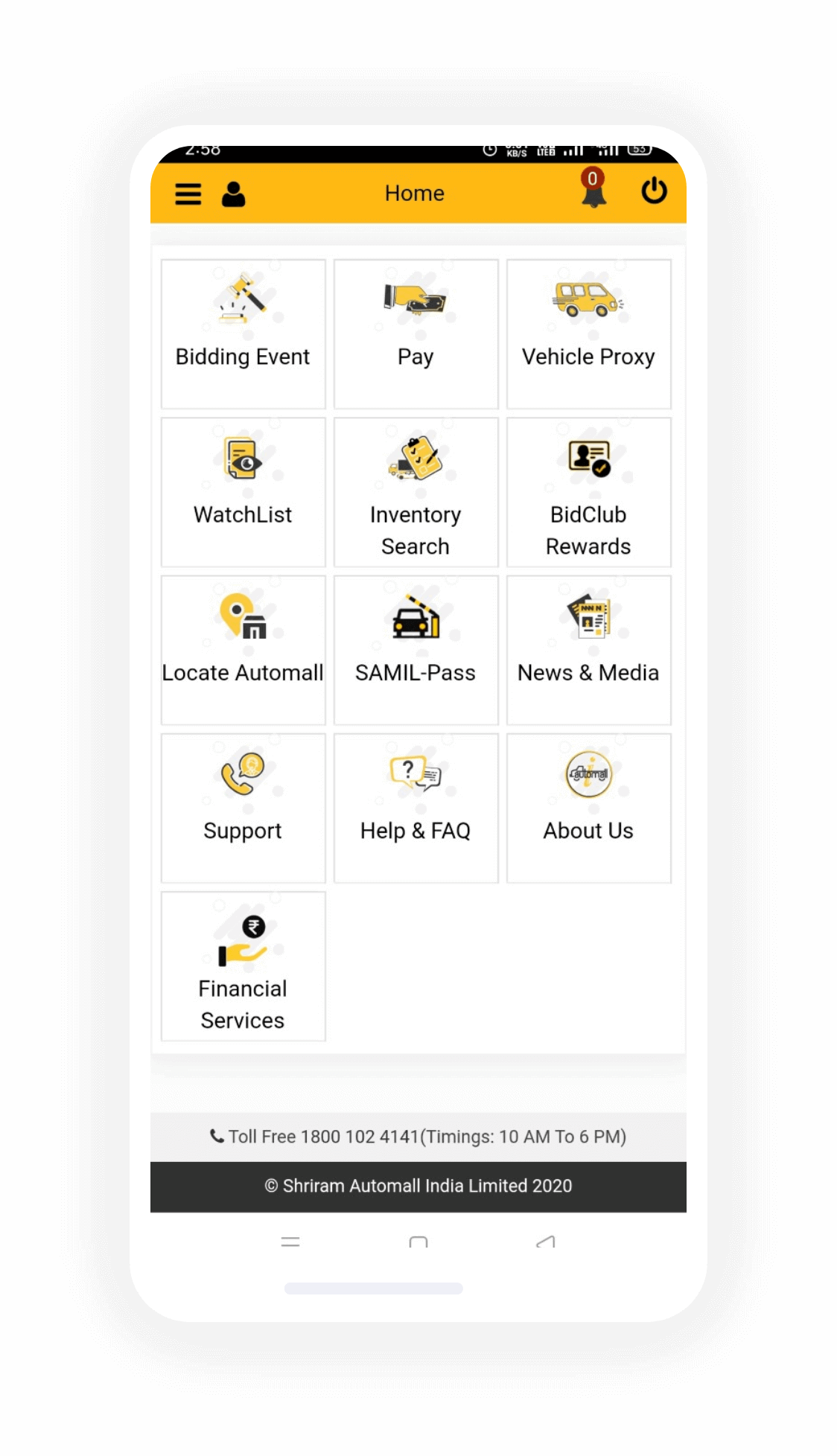This image depicts a smartphone app interface with a predominantly white background. At the very top, there's a yellow horizontal bar with "Home" prominently displayed in the center. To the left of this bar is a menu icon represented by three horizontal stripes, and to the right are two more icons: a bell with a red notification badge marked with a "0" and a power button. Additionally, a small person icon likely representing the user account is situated nearby.

Centrally, the app showcases several clickable options, each enclosed in a square with a yellow icon above it. These options include "Building Event," "Pay," "Vehicle Proxy," "Watch List," "Inventory Search," "Bid Club Rewards," "Locate Auto Mall," "SAML Pass," "News and Media," "Support," "Help and FAQ," "About Us," and "Financial Services."

At the very bottom of the screen, contact information is provided in a structured format. A toll-free number, 1-800-102-4141, is listed, specifying availability hours from 10 a.m. to 6 p.m. Underneath, within a black rectangle, the brand name "Chiram Auto Mall India Limited 2020" is displayed, indicating that this app is likely associated with Chiram Auto Mall, presumably facilitating car sales or rentals.